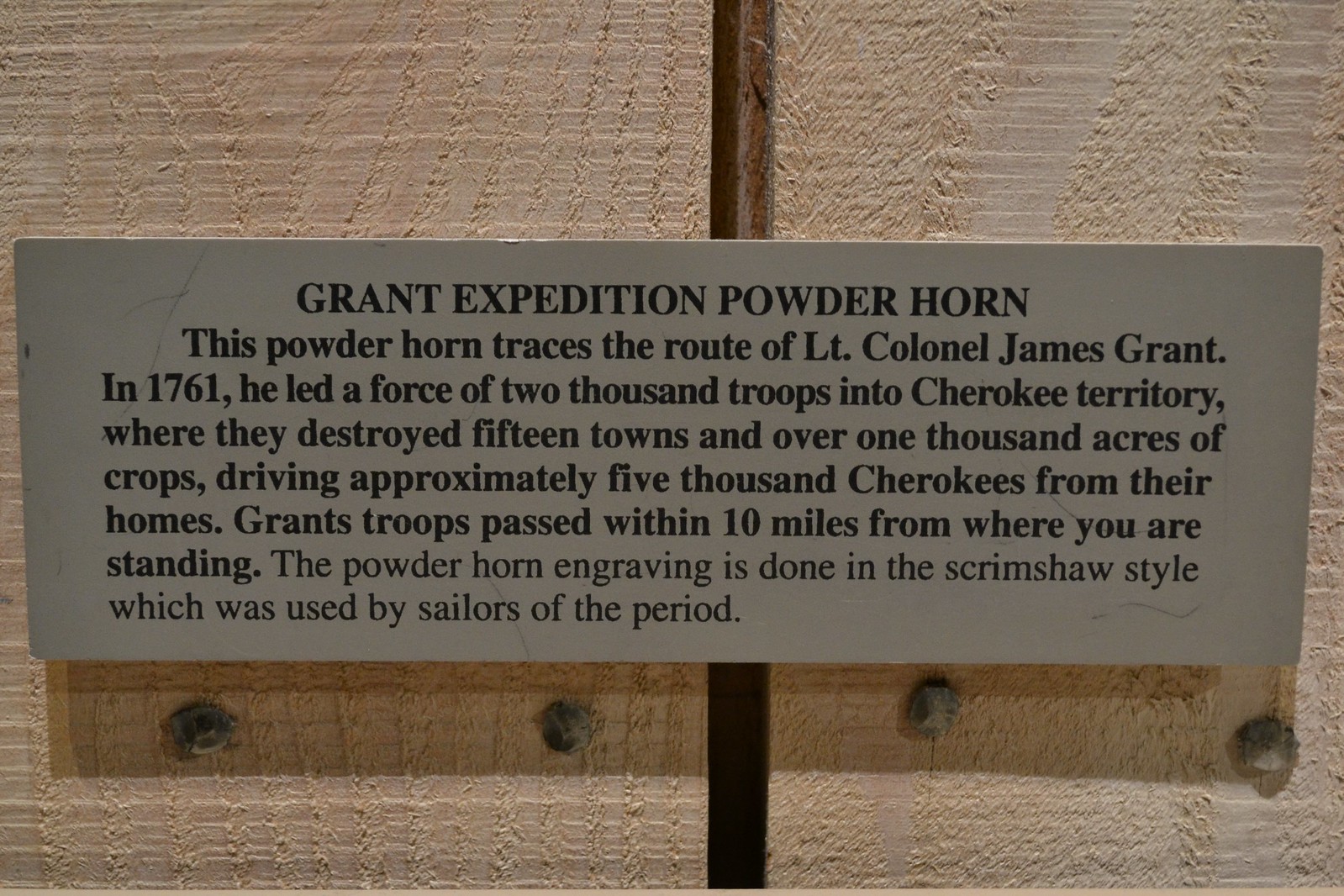The image is a close-up digital photograph of a placard mounted on a split wall held together by two nails on either side. The placard is rectangular and light gray with text in black. The topmost text, in all capital letters, reads “GRAND EXPEDITION POWDERHORN.” Below, in a regular font, it states that this powderhorn traces the route of Lieutenant Colonel James Grant in 1761. He led a force of 2,000 troops into Cherokee territory, where they destroyed 15 towns and over 1,000 acres of crops, driving approximately 5,000 Cherokees from their homes. The plaque notes that Grant’s troops passed within 10 miles of the current location of the viewer. The engraving on the powderhorn is done in the scrimshaw style, traditionally used by sailors of that period. The overall color palette of the image includes tan, silver, and black.